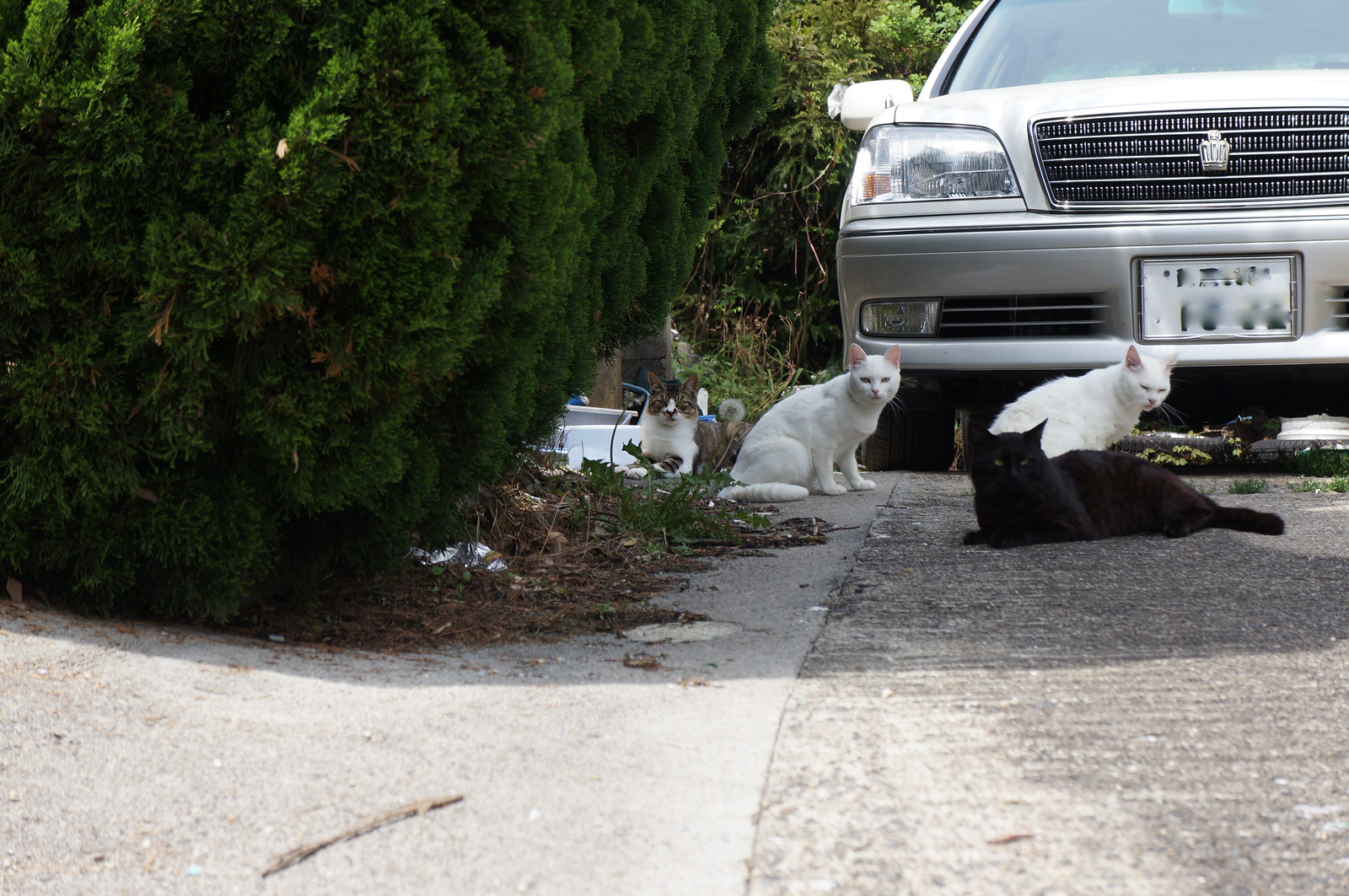This color photograph, taken from a low angle as if the photographer were crouching, captures a scene of four cats lounging on a smooth concrete driveway adjacent to a rougher edge, possibly a sidewalk. To the left, green shrubbery, potentially cypress bushes, partially obscures the view. Behind the cats, the grill of a silver sedan is partially visible, with its license plate blurred for privacy.

In the foreground lies a pure black cat with green eyes, ears perked, and tail curled behind. This cat faces the camera, creating a direct line of sight. Behind the black cat, two white cats sit on their haunches facing to the right. One of these white cats looks forward, directly towards the camera, while the other glances down slightly, its ears attentive. To the left, under the shade of the bush, a gray and white tabby cat with a white patch on its nose lies near the car’s wheel, crouched and staring straight at the camera with a hunted, guilty expression. This cat's distinct posture sets it apart, adding tension to the tranquil setting shared by the other felines.